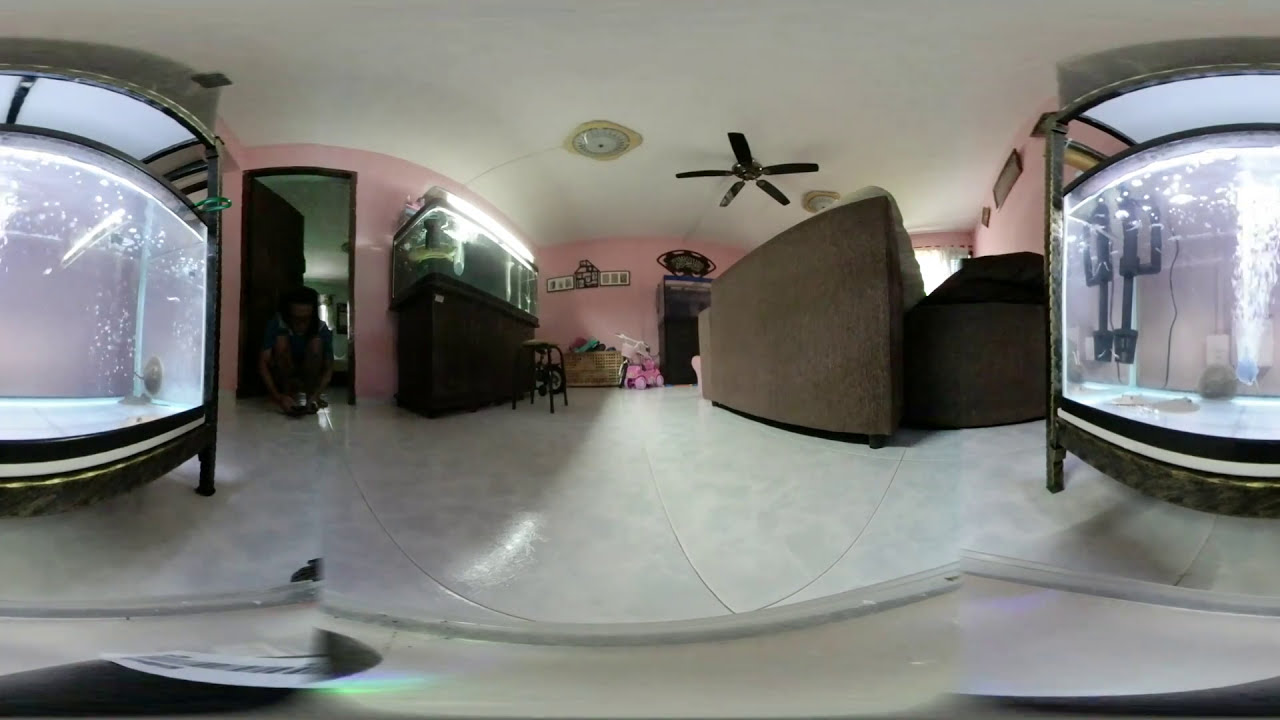The panoramic indoor image captures what seems to be an office area, though the distorted perspective makes some details challenging to discern. Prominently, there are aquariums on both the left and right sides of the room, and due to the lens distortion, the left aquarium might be a mirrored image of the right. Both aquariums exhibit bubbles and lights but no visible fish, except for a single fish spotted in one aquarium towards the center. The room has pink walls that are clearly visible throughout the scene, contrasted by the shiny white tile flooring and a white ceiling with dark brown ceiling fan and lights.

From left to right, the details unfold starting with a person squatting near the left aquarium, next to an open doorway framed in dark brown wood, leading into another room. Moving to the middle of the room, there is a low cabinet or shelf with what seems to be green and red clothing, and adjacent to it are pink objects. A solid brown room divider is observed to the right of this setting, further right is an even darker room divider. Alongside these elements, there's a couch, where only the leg and back are visible due to the low camera angle.

At the far end, centrally positioned, a chest or container is situated, apparently holding some toys on top. To the top right, light seeps through a window, suggesting the photo was taken during daytime. Finally, there's an aquarium on the left side again, this one topped with a large horizontal light fixture. The composite of these items suggests a well-lit, meticulously detailed space, though the exact purpose of some objects and the precise layout remain somewhat ambiguous due to the distorted perspective.